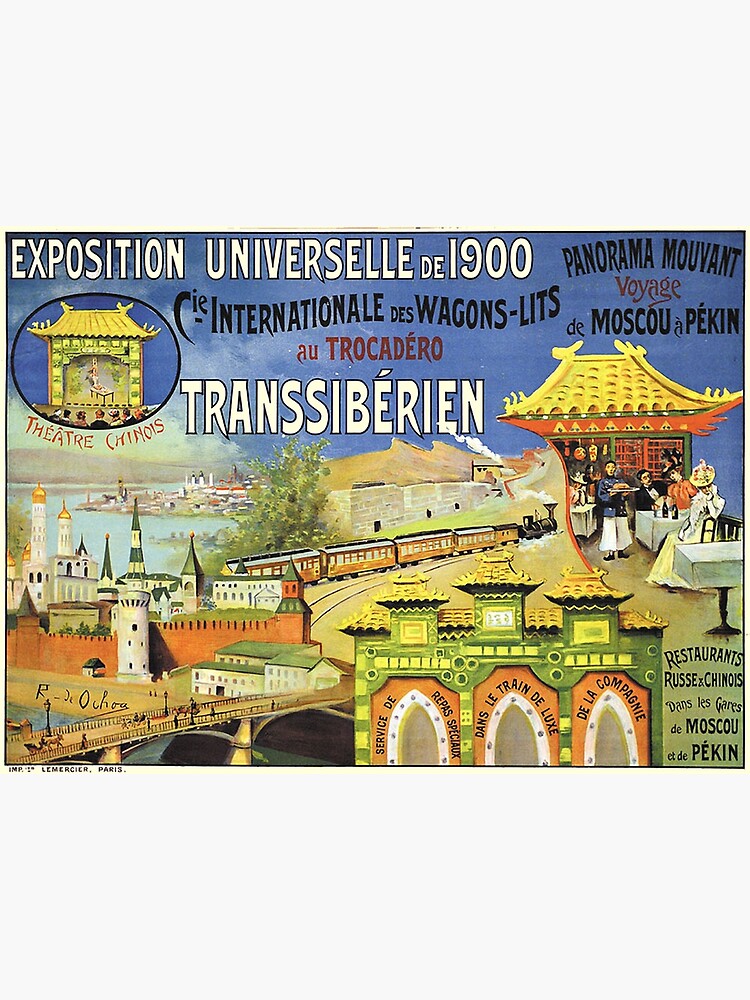This detailed promotional image, likely a poster, is titled "Exposition Universelle de 1900, Trans-Siberian." It showcases a colorful and intricate panorama of the World Exhibition, highlighting various pavilions, emphasizing the fusion of Asian and European architectural styles. On the right-hand side, there is an Asian-style pagoda with a bright yellow, sloped convex archway roof, adorned with a red underside. In front of the pagoda, a dining table is set out, with a waiter holding a platter, ready to serve. Below, in the center, a black train with yellow carriages runs through the middle of the scene, symbolizing the Trans-Siberian Railway.

The background features a diverse cityscape: to the far left, there's a distant city silhouette, while the front left showcases a bridge bustling with pedestrians and a horse-drawn buggy. A green building with yellow convex roofs and white archways, described as offering various services, such as special dining, theater, and deluxe train companies, is located in the bottom right corner. The text throughout the image, mostly in French, includes phrases like "Exposition Universelle de 1900," "International des Wagons-Lits," "Trocadéro Transsibérien," and highlights like "Théâtre Chinois," "Panorama Mouvant," and "Voyage de Moscou et Pékin," enhancing the global and cultural theme of the exhibition.